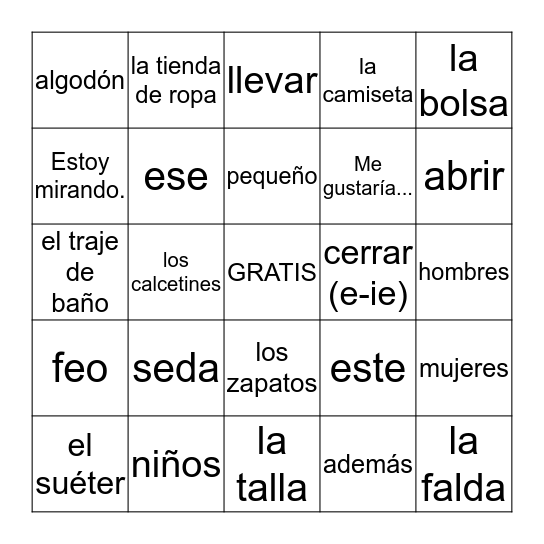The image features a chart with a completely white background and a black outline, arranged in a grid pattern with five columns and five rows, forming a larger square structure akin to a bingo board. Each of the smaller squares within the grid contains Spanish vocabulary words written in a black sans serif font. The font size and boldness vary, with some words appearing in all caps. A couple of the words have "la" or "L" in front of them, and one of the squares includes text in parentheses, although its purpose is unclear.